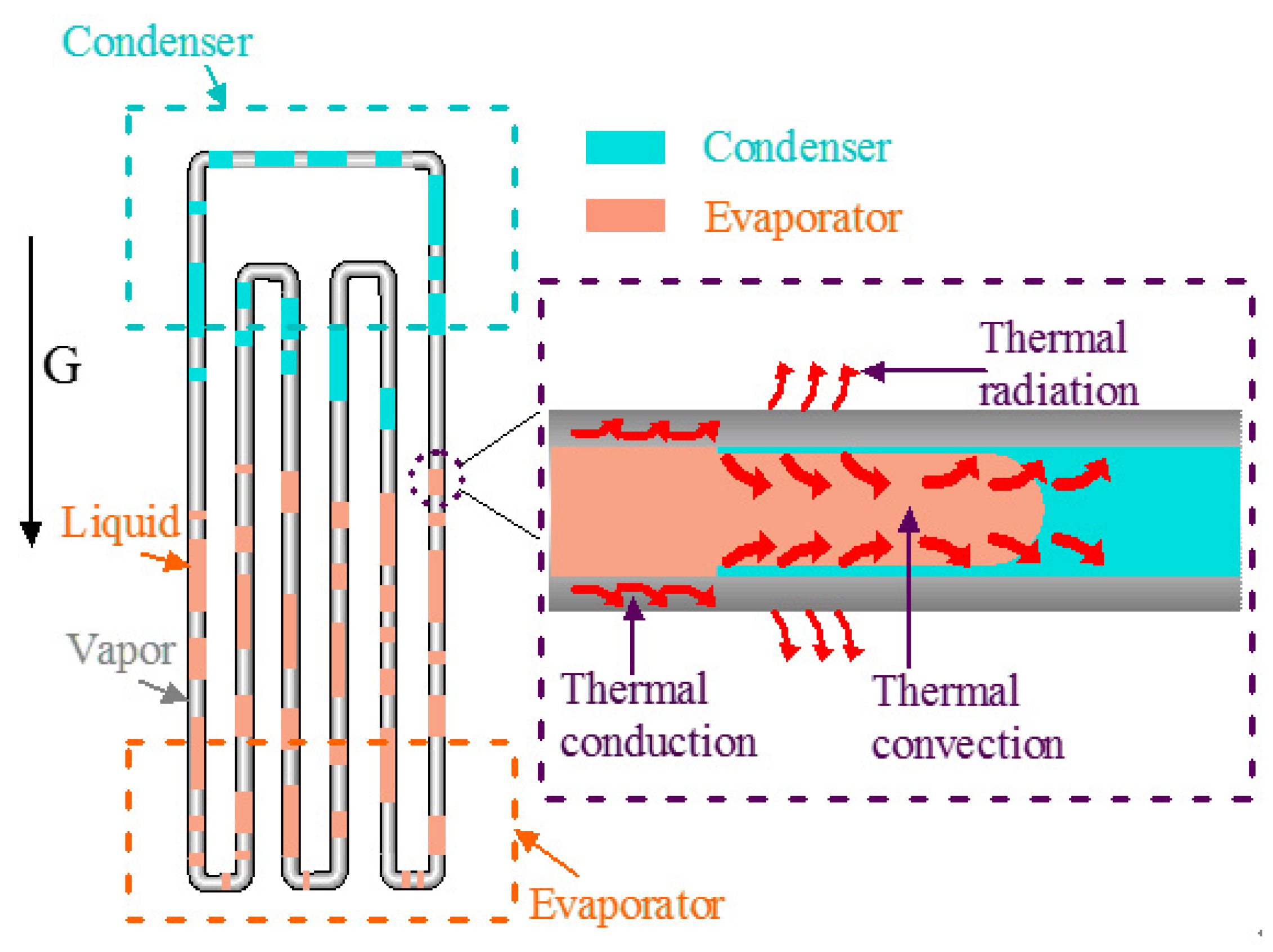This detailed scientific illustration appears to be a diagram of a thermal exchange device, likely an air conditioner, showing the processes of condensation and evaporation. The image is divided into two main sections. The first component features a rectangular arrangement of metal tubing, coiled tightly, representing the inner workings of the device. The top of this rectangular tubing is labeled "Condenser" in bluish-green, while the bottom is labeled "Evaporator" in light orange. Light green and light orange colors indicate the flow of liquids and vapor within the tubes, with blue lines marking the condenser parts and red lines marking the evaporator.

In the center of the illustration, there is a prominent downward-pointing black arrow labeled 'G,' likely denoting gravity. Small pink dots and pink arrows labeled "Liquid," along with gray arrows and text labeled "Vapor," indicate the phases of the substance transitioning through the tubing system.

The second part of the diagram extends horizontally from left to right and provides a detailed view of different types of thermal processes occurring within the device. This section is marked with black arrows and labels identifying "Thermal radiation," "Thermal convection," and "Thermal conduction."

Overall, this diagram comprehensively illustrates the mechanisms of thermal exchange, emphasizing the roles of the condenser and evaporator, and highlights the importance of thermal dynamics in such a system.